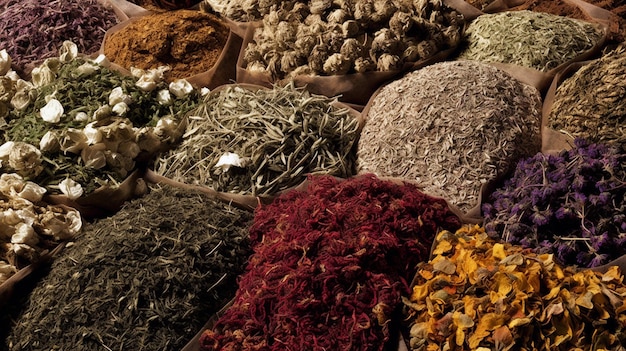The photograph captures an up-close view of an array of colorful herbs and spices meticulously arranged in short, brown cardboard or canvas containers, evocative of a bustling spice market in places like Morocco or the Middle East. The display features approximately twelve distinct piles of herbs and spices, creating a vibrant mosaic of colors including purple, yellow, red, green, tan, golden, beige, and brown. Each container holds a unique blend of dried ingredients, some finely ground and others in more substantial forms, suggesting diverse culinary or homeopathic uses. The perspective of the photograph is slightly elevated, offering a comprehensive view of the orderly rows of spices, which are organized in three rows with four piles in each. Notable details include a green pile with what appear to be white petals, hinting at the variety’s potential use as a tea or remedy. The overall composition vividly conveys the rich sensory experience typical of traditional spice markets.